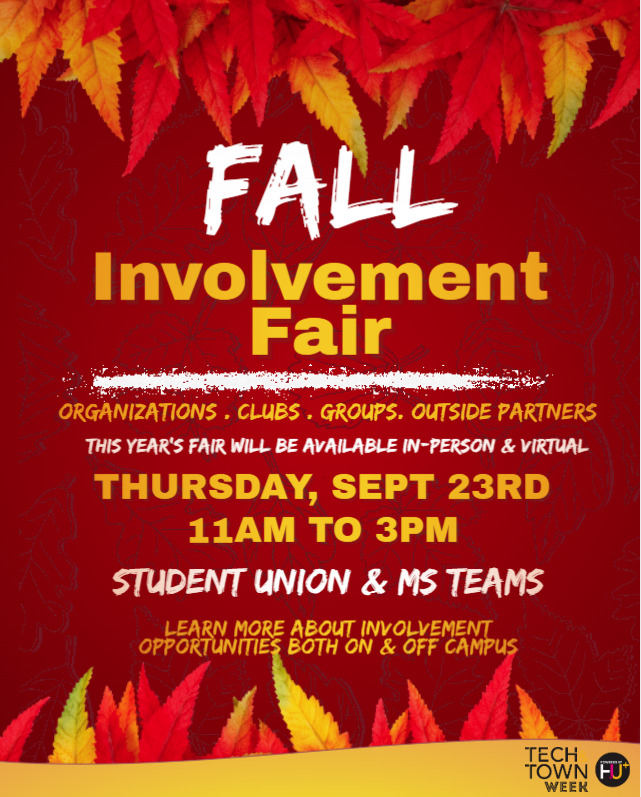This poster for the Fall Involvement Fair features a predominantly dark red maroon background adorned with vibrant autumn leaves at the top and bottom. The leaves are primarily yellow and red, with some green accents scattered amongst them. At the top of the poster, large white letters spell out "FALL," below which "Involvement Fair" is written in bold yellow letters. 

In the center, a splash of white paint with dotted edges runs across the poster, overlaid by the words "Organizations, Clubs, Groups, Outside Partners" in gold-yellow. The poster announces that this year's fair will be available both in person and virtually, detailed in white text. Key event details are prominently displayed in yellow: "Thursday, September 23rd, 11 a.m. to 3 p.m.," followed by the venues "Student Union" and "MS Teams" in white.

Towards the lower right corner, "Tech Town Week" is noted in a light gold band, accompanied by a circular logo with an "F" in white and a colorful "U." This elegantly designed poster, slightly taller than it is wide, invites students to explore various involvement opportunities on and off campus, capturing the essence of the fall season with its harmonious blend of colors and detailed informational layout.